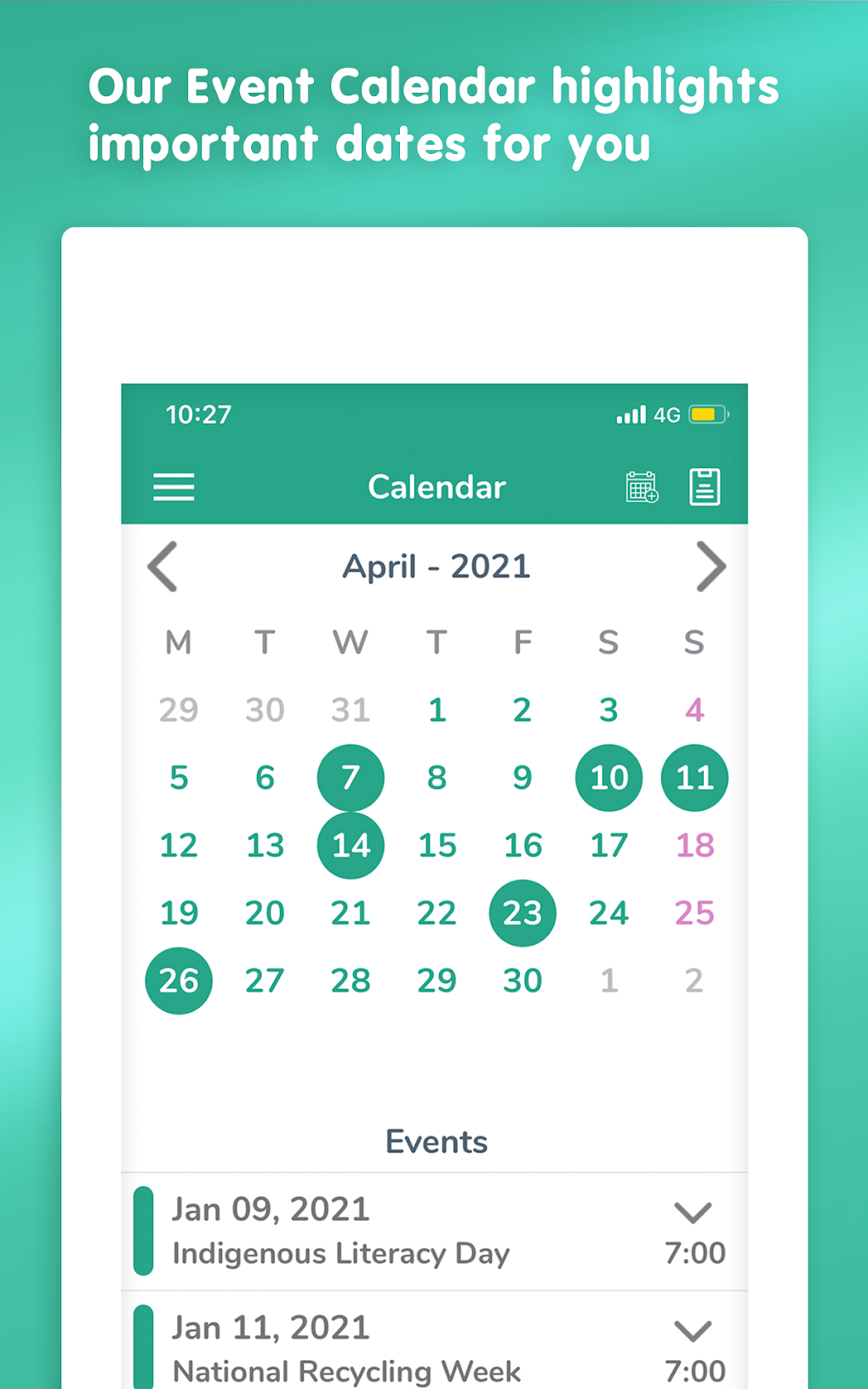**Event Calendar Screenshot - April 2021**

The screenshot captures an event calendar with a teal and white color scheme, accentuated by light lavender highlights. 

At the top of the screen, a teal banner features the text "Our Event Calendar highlights important dates for you" written in Comic Sans font with white lettering. Above this banner, the device status bar displays the time as 10:27, along with four signal bars indicating 4G connectivity, a battery symbol, and a three-line menu icon, known as a hamburger menu.

Below the banner is the main calendar section, starting with a teal header labeled "Calendar." Immediately beneath, it shows the month and year, "April 2021," flanked by navigation arrows allowing the user to move to previous or following months.

The calendar grid starts the week on Monday (M) and includes day headers M, T, W, T, F, S, S. Dates from the previous month (March 29th, 30th, and 31st) are displayed in gray. The current month's dates are in teal, beginning with Thursday, April 1st, and extending through Friday, April 30th. Gray dates marking the start of the next month, May 1st and 2nd, are also visible.

Beneath the calendar, there is a section titled "Events" with details of two highlighted events:

1. **Indigenous Literacy Day** on January 9th, 2021, at 7:00 PM.
2. **National Recycling Week** on January 11th, 2021, at 7:00 PM.

This detailed event calendar provides a clear and visual way to keep track of significant dates and upcoming events for the month of April 2021.